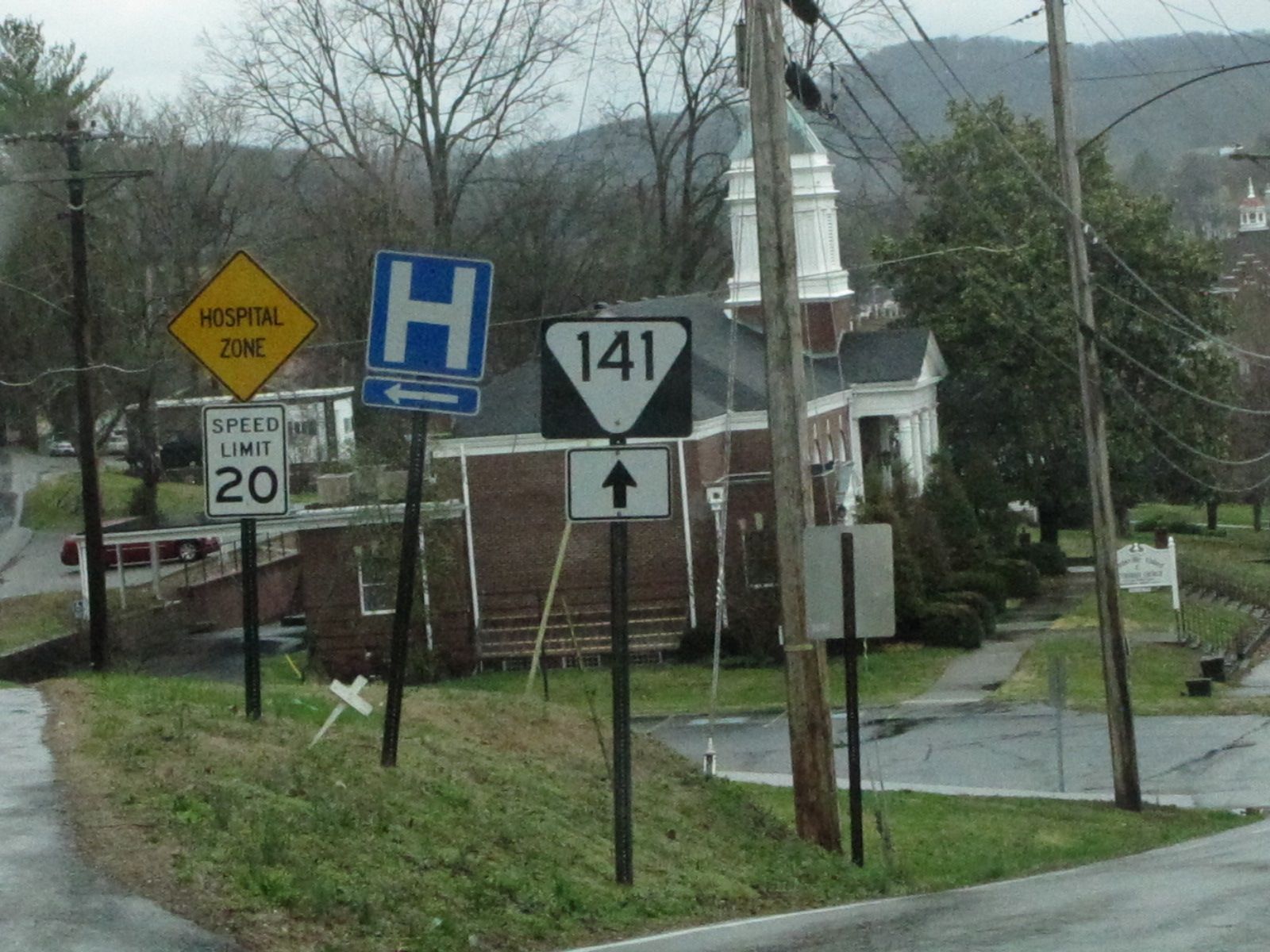Image Caption: 

Nestled in a serene countryside setting, the image showcases a charming brown house adorned with distinctive white and green stipple accents. The house is situated on a lower portion of sloped land, surrounded by lush green vegetation and gentle hills in the background. In the foreground, positioned on a higher slope, multiple road signs are visible. The signs include an orange diamond-shaped "Hospital Zone" warning, a white rectangular "Speed Limit 20" notice, a blue "H" sign indicating the direction to the hospital, and a highway sign labeled "141" marking a specific route. Power lines stretch across the landscape, adding a touch of modern infrastructure to the rustic scenery.